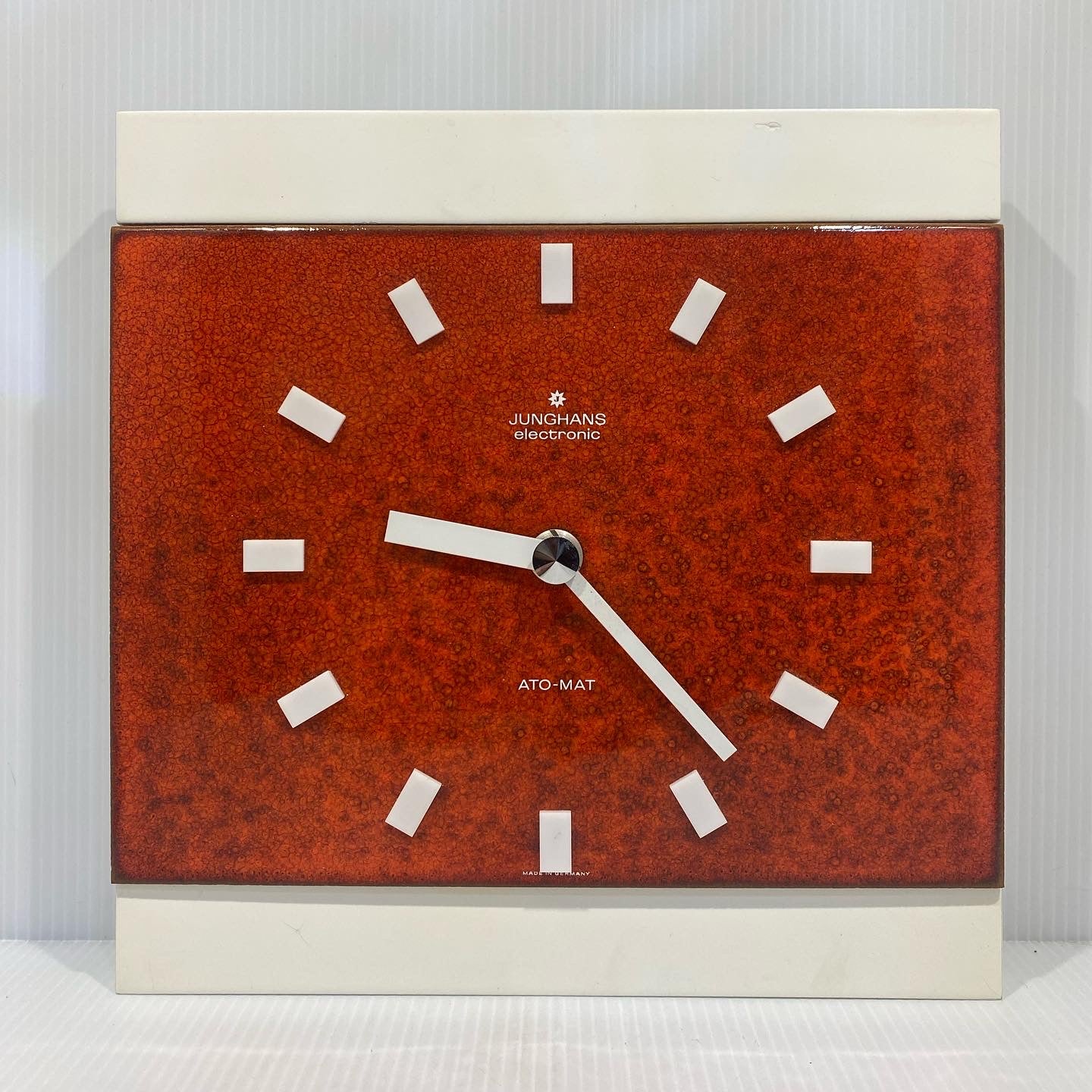The photograph showcases a square, burnt orange analog clock, set against a white background with a gray wall and white floor in the backdrop. The clock, primarily focus of the image, features cream-colored borders at the top and bottom, enclosing a central red rectangle. It has white rectangular hash marks indicating the hours, and white analog hands. Below the 12 o'clock mark, the text reads "Jung Chan's Electronic," and above the 6 o'clock spot, it says "Automat." The clock displays the time 9:23 and is equipped with small, silver, rectangular buttons for setting the time.